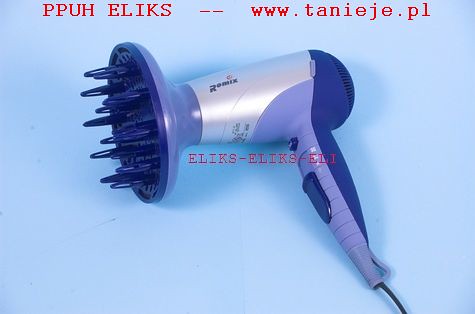This photograph features a uniquely designed device resembling a hairdryer, set against a light blue background. The device has a base of silver with purple and dark blue accents— the handle is primarily silver with dark blue switches, while the head is dark navy blue. Instead of a regular nozzle, it has a circular disc at the front with black plastic spikes protruding from it, suggesting it may serve as a massaging or relaxation tool.

The image appears to be a product shot, illuminated by multiple light sources as evidenced by the shadows surrounding the device. At the top of the photograph, there is prominent red text displaying "PPUHLX" followed by double hyphens and the website "www.tanieje.pl". This text partially overlaps with the object but is mostly clear against the background. In the middle of the image, superimposed in smaller red text, are the letters "ELIKS-ELIKS-EL1 or I", acting as a watermark.